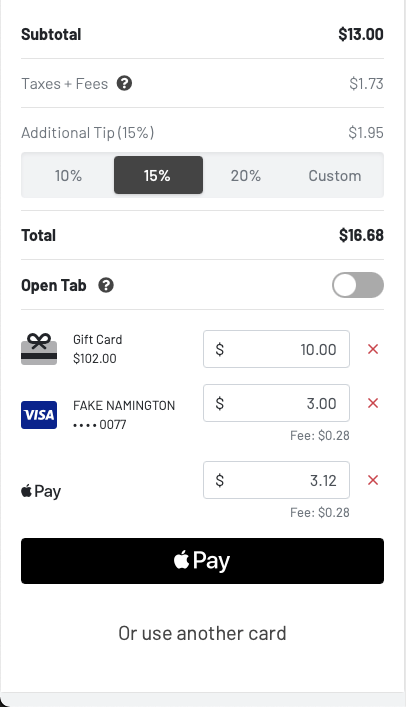This is a detailed screenshot of a digital receipt. On the left side, there is a subtotal listed in bold black letters amounting to $13.00. Below the subtotal, "Taxes and fees" are noted, next to a question mark enclosed in a circle, totaling $1.73. An additional 15% tip equates to $1.95. The grand total is $16.68. 

The option for an open tab is toggled off. There is a gift card used for $10.00, marked with an 'X' for potential modification. Then, a Visa card under the name "Fake Namington" is used for $3.00, which incurred a $0.28 fee—this Visa amount is highlighted in blue while all other text remains in black. Apple Pay is used for the remaining $3.12, also marked with an 'X'. 

The overall layout has all elements on a white background, and a note is present indicating the possibility of using another card.